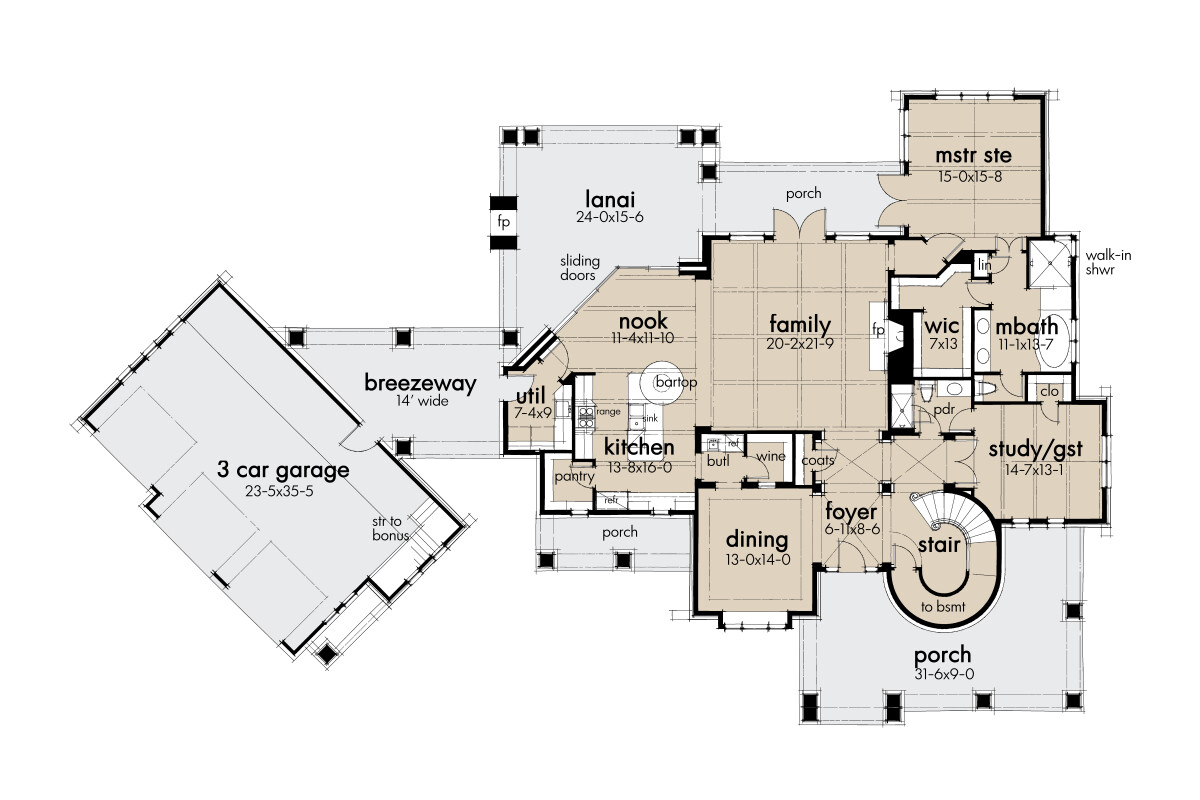The image depicts a detailed blueprint of an expansive mansion, viewed from above, showcasing all the rooms and structural elements in a light gray and light brown color scheme. The blueprint features a three-car garage located on the left side of the image, connected to a breezeway. This breezeway leads to a utility room, which in turn opens into a nook adjacent to the kitchen. The kitchen extends into a large family room, with a fireplace and a porch access. Adjacent to the kitchen is a distinct dining area connected to a butler area and a wine storage space, leading towards a foyer with circular stairs ascending to the second floor. The main floor includes a master suite positioned in the upper right-hand corner, complete with a master bathroom, walk-in shower, and walk-in closet. The suite also opens onto a porch area. Additional rooms on this level include a study guest room with a closet and a bathroom. The layout is designed to seamlessly integrate living spaces with non-living areas, offering a spacious and functional living environment.